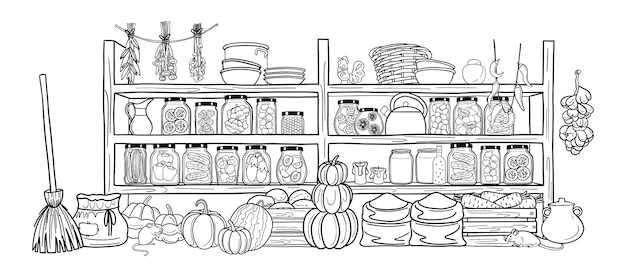This detailed black-and-white sketch depicts an old-school pantry reminiscent of a Fantasia-era setting, brimming with an array of items and fine details. On the left side of the scene, an upright straw broom leans against an invisible wall. The floor, which appears to be adorned with stone, is filled with various produce and supplies: multiple sacks of flour, whole pumpkins and gourds, three of which are prominently stacked atop one another, watermelons, and a wooden crate filled with carrots. Two mice scurry across the floor; one by the pumpkins and the other near the crate of carrots.

The background features a set of two large, subdivided wooden shelves filled with an eclectic assortment of pantry goods and utensils. Hanging herbs and garlic add to the rustic charm, dangling from the left side of the shelves. The top shelves are adorned with baskets, a wicker basket with additional baskets in front of it, drying peppers, a chicken statue, pots, pans, and other boiling utensils. 

Below, the middle shelves house various glass jars, pitchers, and a tea kettle, as well as jars of different sizes filled with pickled vegetables such as eggplants, peppers, tomatoes, and pickles, some with black lids. The assortment continues with more rounded glass containers filled with preserved fruits and vegetables. Charming details include a pair of candles and a small jug with handles on the lower shelves.

Overall, this intricate sketch captures the essence of a bustling, well-stocked pantry in a timeless, enchanting universe.